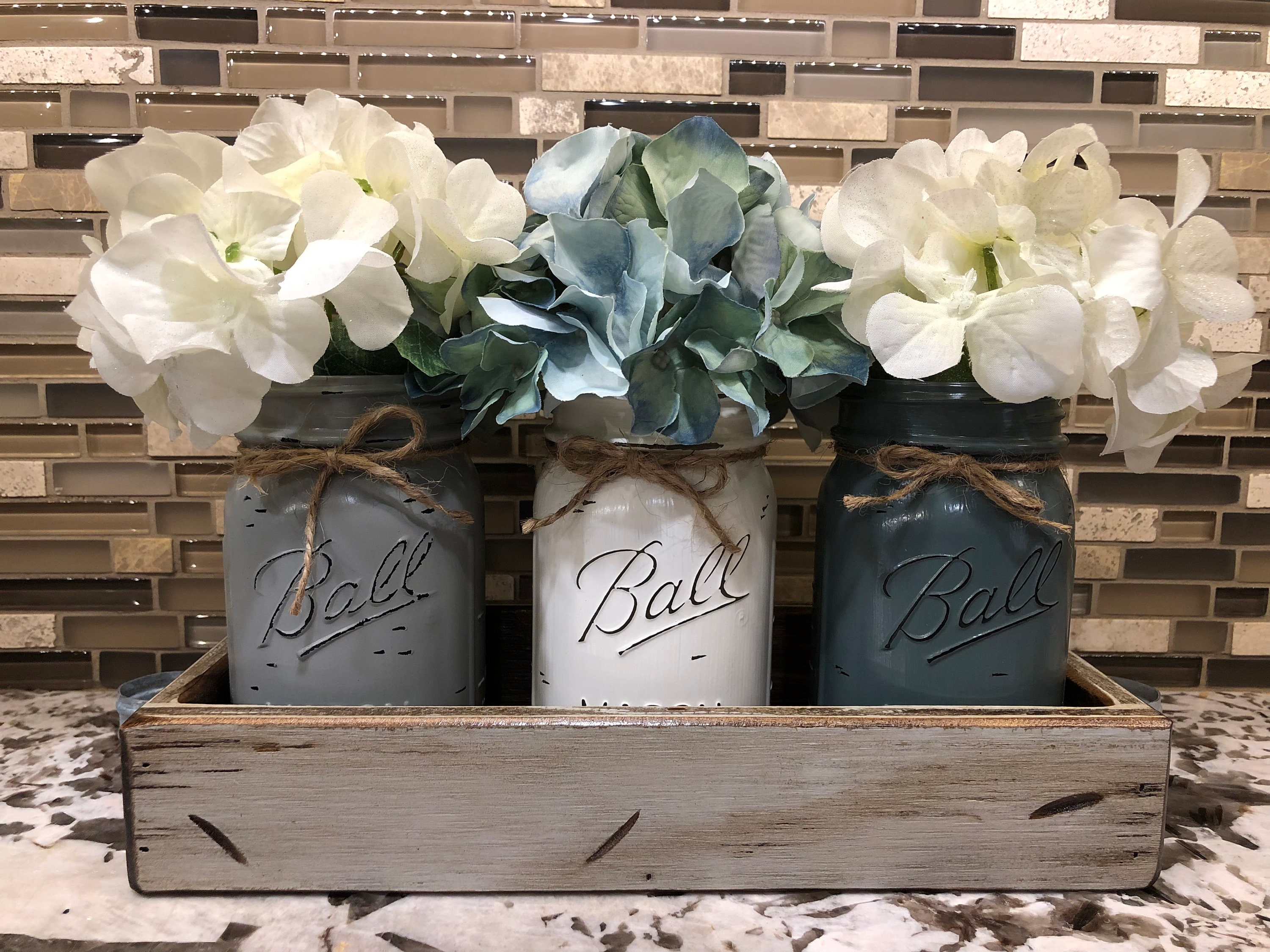This is a close-up color photograph of a farmhouse-style kitchen counter decorated with a charming arrangement. Centered on the marbled white and brown countertop is a light brown wooden tray holding three Ball mason jars, each of which has been chalk painted in different colors: gray on the left, white in the middle, and dark forest green on the right. Each jar is adorned with a piece of brown craft twine tied into a bow around its neck. The jars are filled with faux hydrangeas; white flowers on the outer jars and bluish-white flowers in the middle jar. These decorations are set against a modern, multicolored tile backsplash featuring a mix of brown, white, tan, and gray stones, adding an elegant yet rustic touch to the kitchen space. The overall color palette of the scene is muted and harmonious, incorporating earthy browns, blues, and grays.